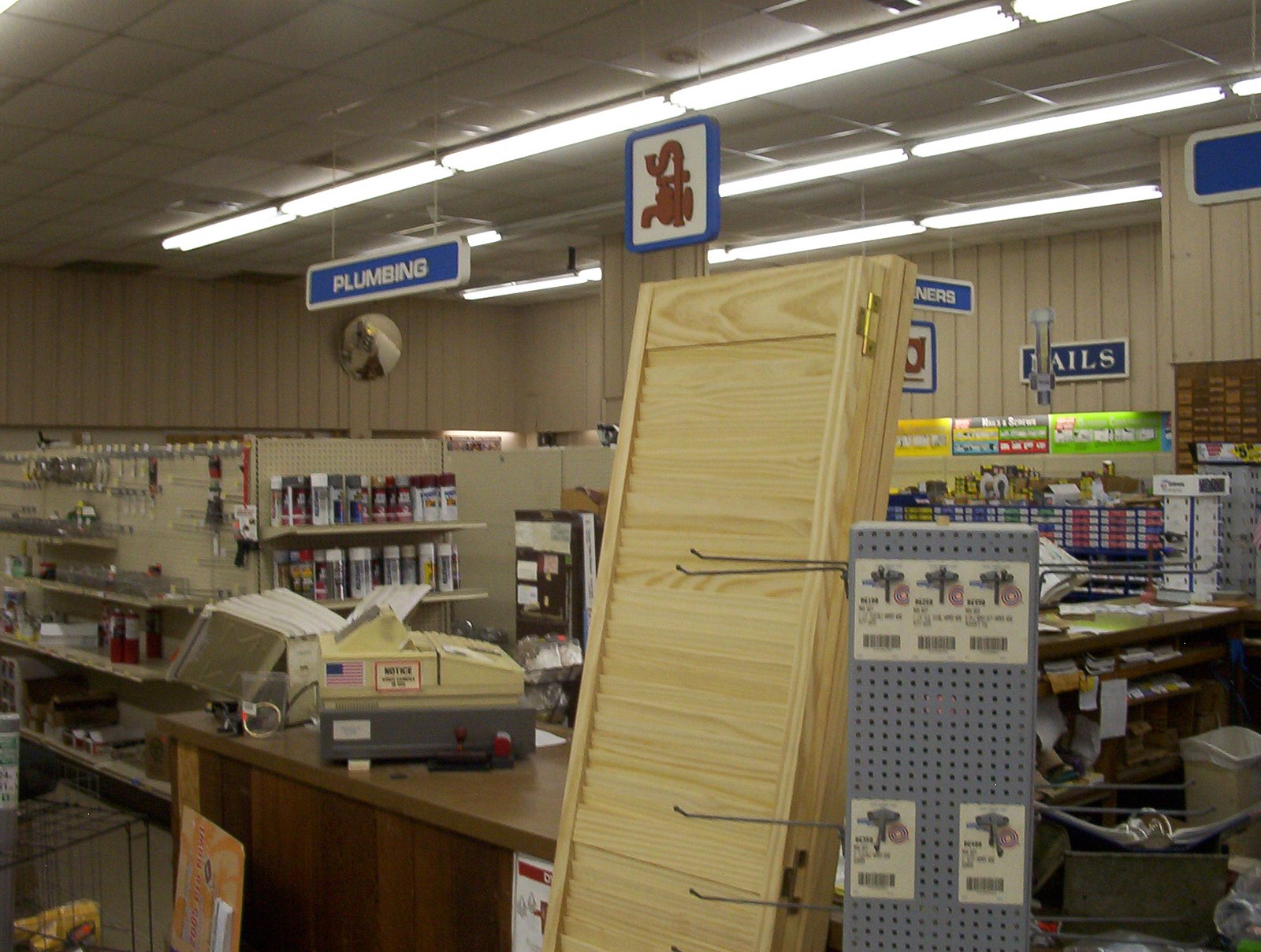This is a detailed photograph of an interior corner of a hardware store. Dominating the upper left corner of the image is a sign with the word "plumbing" written in white, indicating the store's plumbing section. Beside it is a vertical rectangular sign featuring a picture of a pipe to facilitate visual shopping. The centerpiece of the scene is an old cash register adorned with an American flag sticker and another sticker labeled 'notice', though the smaller text is illegible.

To the right of the register, the image captures two tiers of shelves packed with various cans of spray paint. These cans are predominantly white, silver, red, some with yellow accents, adding a splash of color to the setting. In the distant background, blue shelving lined with innumerable tiny drawers labeled 'nails,' 'nuts,' and 'screws' are spotted, catering to the store's organizational needs. Supporting the back section's signage are small wooden drawers, presumably for sorting these individual pieces.

In the far-right foreground stands a gray pegboard with an assortment of papers glued to it, their content indiscernible. Below this pegboard, shelves under a counter appear cluttered and disorganized, clearly indicative of the working area behind the counter. Nearby, leaning wooden doors – possibly intended as room dividers – are hinged together, suggesting versatility in store layout. Adding a subtle artistic touch to this utilitarian environment is a painting of a city skyline, providing a quaint backdrop to the practical hardware offerings. Across from the register, distinct shelves organized with toolkit essentials further confirm the store's comprehensive range of hardware supplies.